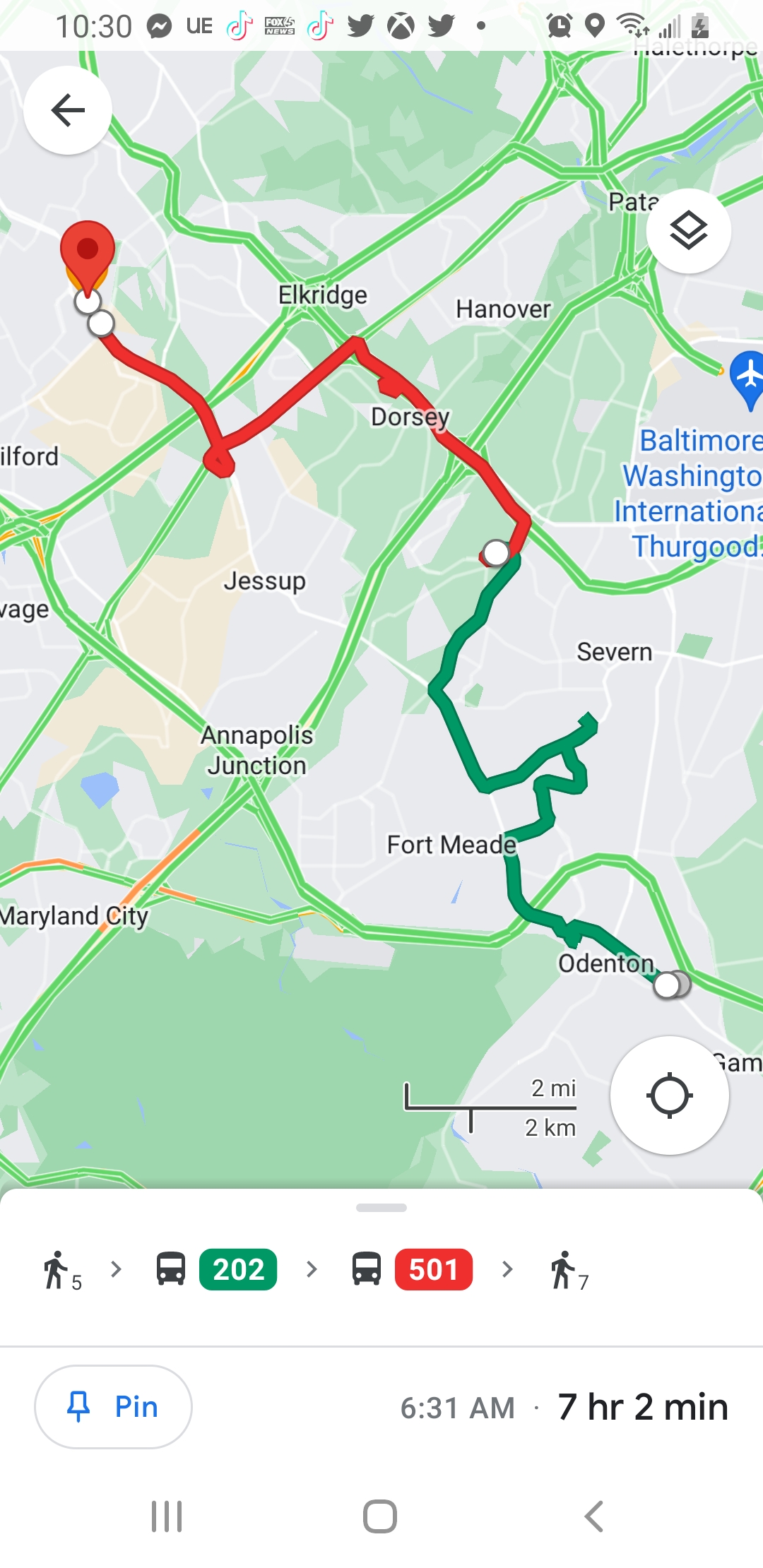This detailed caption accompanies an image of a smartphone screenshot displaying a navigation route on a map application. The app interface is predominantly white, while the map itself is rendered in varying shades of grey, green, blue, and tan. The highlighted path begins in Odenton, located in the bottom right corner of the screen, traverses through Fort Meade, and then meanders upwards in a squiggled pattern toward the middle right. Initially, this route is color-coded in dark green, which then shifts to red midway through. A single white point is illustrated, intersected by the red line that passes through Dorsey in the northwest, continues with some dips and rises, and culminates at the final destination. This endpoint is marked distinctly with two white dots and a red marker. Additionally, the top of the phone screen features various app icons, including two for Twitter, two for TikTok, Xbox, Alarm, among others.